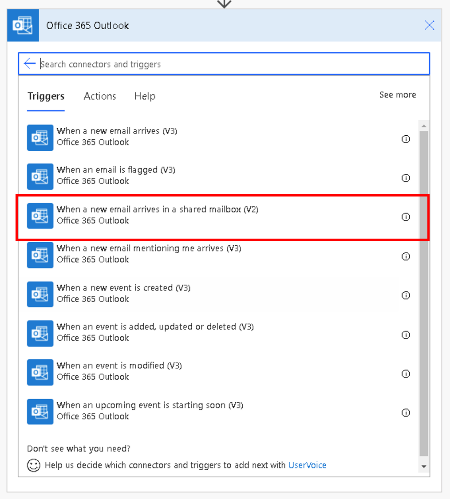This is a screenshot from Microsoft Office 365 Outlook with a thin gray border surrounding the image. At the top, a pale blue bar displays "Office 365 Outlook" in black text. In the upper right-hand corner, a blue "X" icon allows the user to close the window. On the upper left-hand corner, there is an icon resembling a grid pattern.

A blue outlined search box with a back arrow is labeled "Search Connectors and Triggers." Below the search box, three options are presented: Triggers, Actions, and Help. The Triggers option is currently selected, with "See More" on the far right-hand side.

The available triggers listed begin with "When a New Email Arrives V3," followed by "When an Email is Flagged V3." Among these options, the trigger "When a New Email Arrives in a Shared Mailbox" is highlighted with a red box.

The list continues with "When a New Email Mentioning Me Arrives," "When a New Event is Created," "When an Event is Added, Updated, or Deleted V3," "When an Event is Modified V3," and "When an Upcoming Event is Starting Soon V3."

At the bottom of the list, there is a prompt asking, "Do you see what you need? Help us decide which connectors and triggers to add next with User Voice."